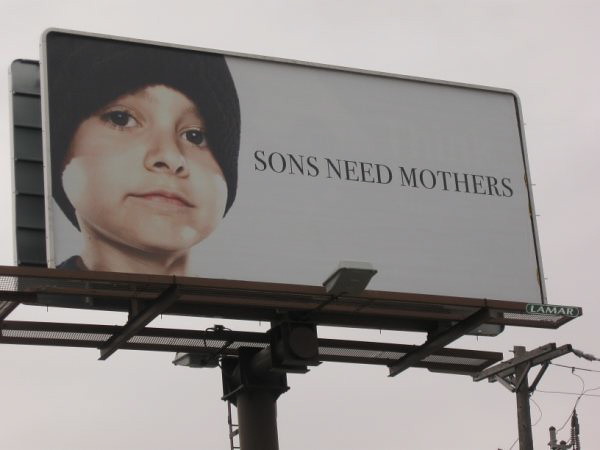This rectangular, horizontally oriented image captures a stark scene under a gray sky. Dominating the center is a large rectangular billboard mounted on a tall pole. The billboard itself has a clean, white background and prominently features the image of a young Caucasian child's face, possibly around five or six years old. The child, with beautiful brown eyes and an adorable expression, wears a dark black beanie hat. To the side of the child's image, the billboard bears a poignant message in large capital letters: "Sons Need Mothers." In the lower right corner of the billboard structure, the name "Lamar" is displayed in white text. The overall atmosphere of the image is somber yet evocative, drawing attention to its important message.